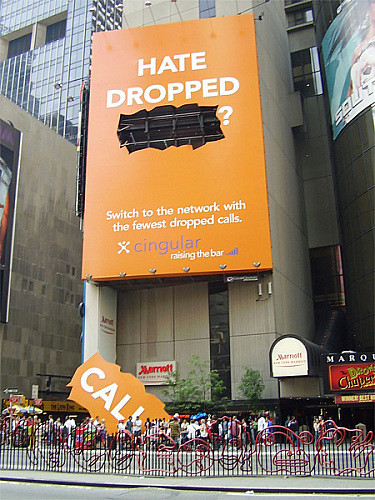The outdoor color photograph, taken from street level on a bright day in the city, focuses on a large vertical rectangular billboard attached to the side of a multi-story light gray skyscraper, which appears to be a Marriott hotel. The billboard, in the upper half of the image, features clever advertising from the cellular company Cingular. The sign, predominantly orange with white capital letters at the top, reads "HATE DROPPED" followed by a question mark. Below it, a die-cut section with the word "CALLS" appears to have fallen out and is now resting on the ground, creating the illusion of dropped calls. Smaller white text below reads, "Switch to the network with the fewest dropped calls," followed by the Cingular logo and the slogan "Raise the bar". The foreground shows a busy street and sidewalk with people walking and standing, some seemingly engaged with the billboard. A red wrought iron barricade, possibly decorative, extends down the middle of the street. Additionally, the image captures another orange, diagonally positioned sign which reads "CALL" in white letters. The left side of the image features the skyscraper with light blue windows, enhancing the urban feel of the scene.